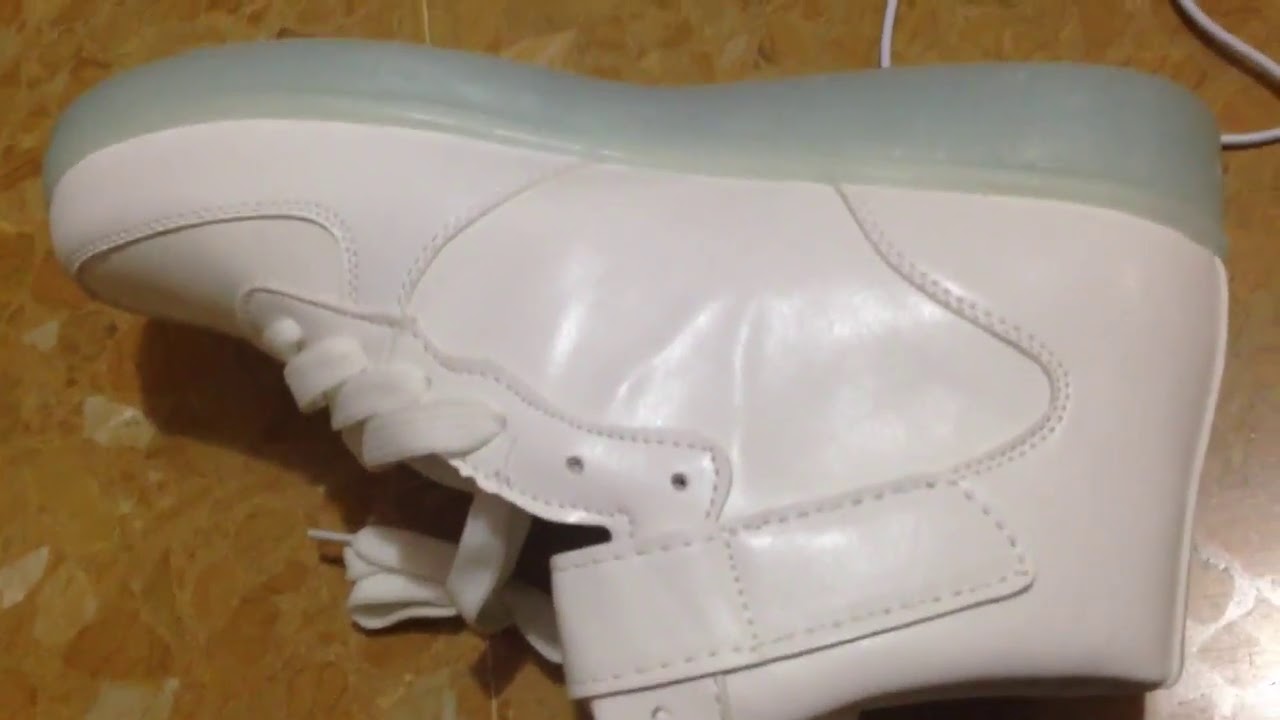The image depicts a small, white child's high-top sneaker, likely resembling a Nike design, lying on its side on a dark tan and white speckled surface, potentially a marble or tile floor, or a chipboard or wooden surface. The sneaker has white laces threaded through the first four eyelets but not fully laced up, and it appears untied. It features a bluish, semi-transparent heel and visible stitched panel details across the shoe. Additionally, a white cord, similar to an iPhone charger, is seen in the top right corner of the image. The photograph is taken indoors, with light reflecting off the shoe, particularly from the bottom right, emphasizing its central position, and its heel is oriented at the top of the image.